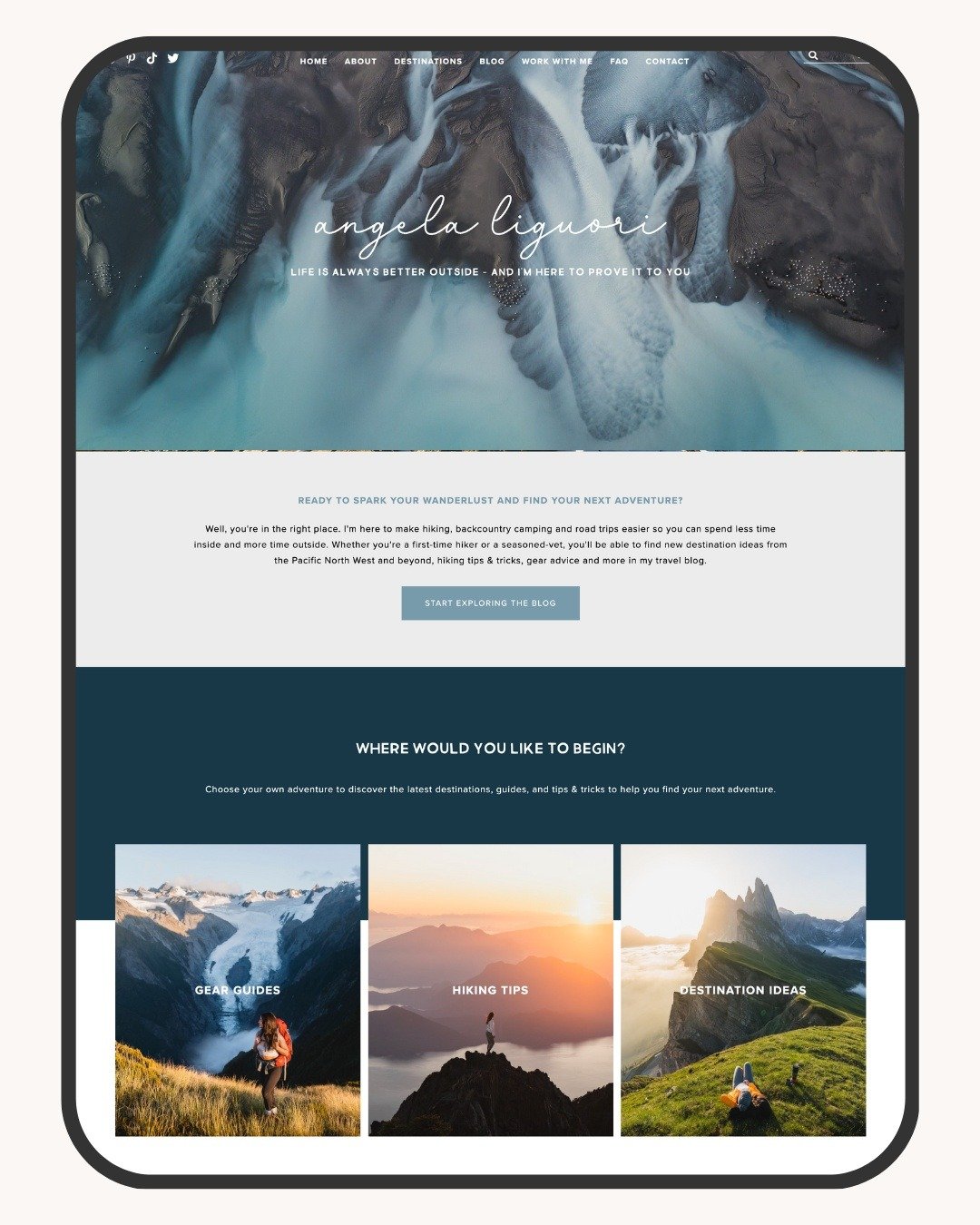The image features a black border enclosing several elements. At the top, a gray, brown, and white image appears, resembling either trees, mushrooms, or perhaps a snowy landscape, though the exact details are ambiguous. Below this, there is a cursive signature reading "Angela [Unreadable Last Name]." A prominent caption states, "Life's always better outside and I'm here to prove it to you."

Further down, the image contains a paragraph of text, though it is mostly blurry and indecipherable, followed by a large blue button. Below the button, a navy blue section asks, "Where would you like to begin?" This section includes a barely legible sentence and features three smaller images beneath it: the first depicts a person walking along the side of a mountain with a glacier visible below; the second shows someone standing atop a mountain during sunset. The third image is not described in the provided information.